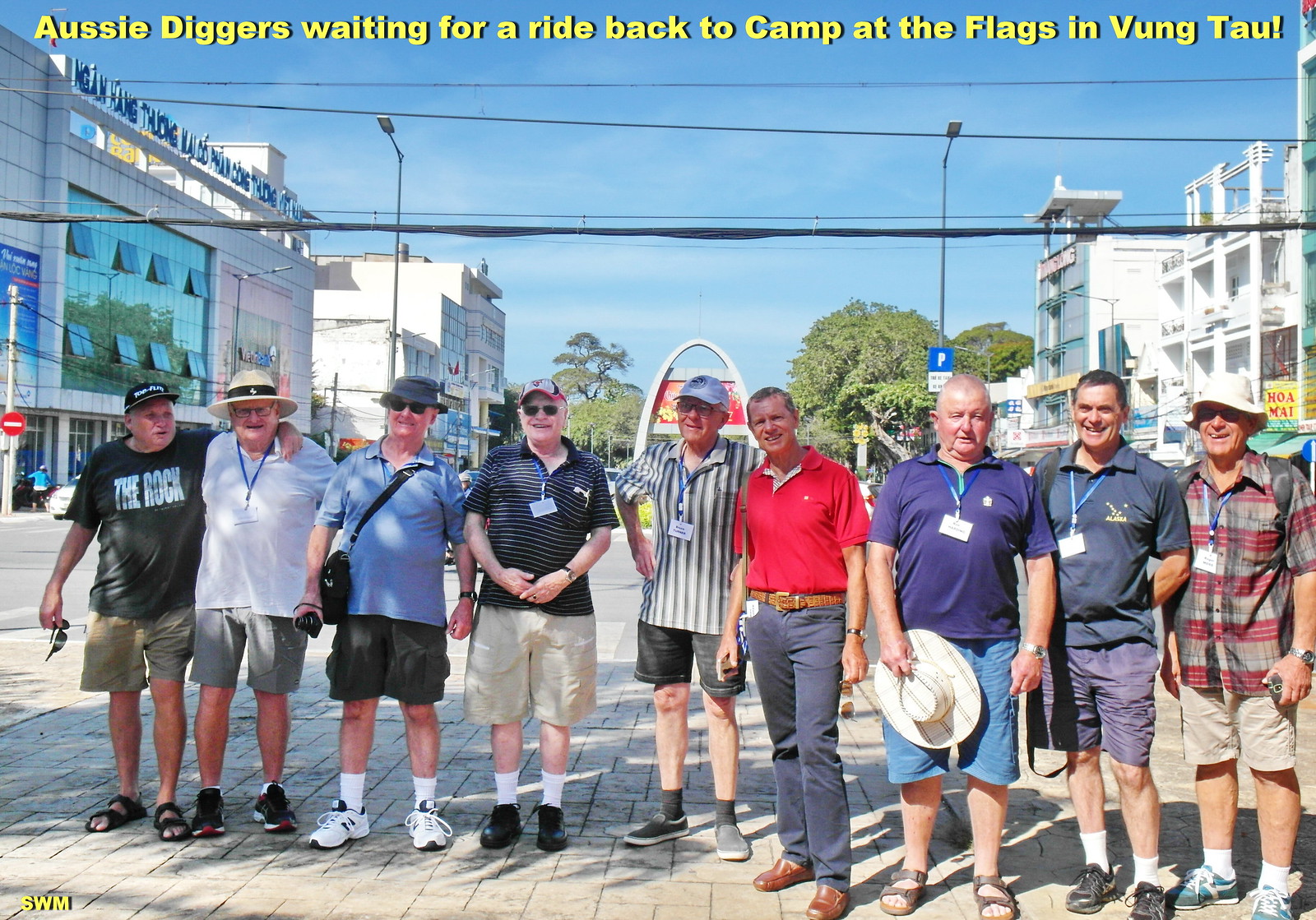This color photograph, captured on a partly cloudy day, shows nine older gentlemen standing shoulder-to-shoulder in a cheerful line outside a town in Australia. All in their fifties, the men are dressed casually in t-shirts, polo shirts, or plaid button-ups, paired with shorts or chinos, and most are wearing sneakers. Many have sunglasses and sun hats or baseball caps, along with blue lanyards likely holding name tags, possibly indicating they are part of a tour group. They are standing in a lively outdoor shopping plaza with storefronts and shops on either side, electric or telephone lines crossing overhead. Behind them, a small silver archway statue adds a distinctive touch to the background. The photo's context is given by the yellow text at the top reading, "Aussie Diggers Waiting for a Ride Back to Camp at the Flags in Vung Tau," and the small yellow "SWM" in the corner at the bottom. The men are all smiling and appear to be enjoying their time together, radiating a friendly camaraderie.